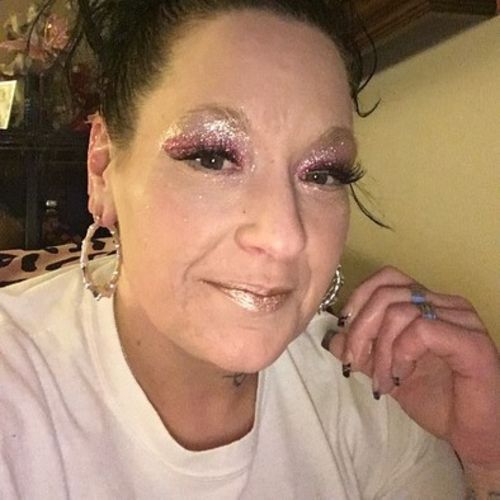The close-up image is of a woman, either white or Latina, with dark hair pulled back into a slick, shiny bun secured with gel or styling product. Her makeup is dramatic, featuring heavy, glittery eyeshadow that layers pink glitter and silver glitter extending up to her eyebrows. She wears false eyelashes and her dark eyes are enhanced by this striking eye makeup. Her lips are adorned with a metallic, peachy-copper shade of lipstick. She accessorizes with large silver hoop earrings and two silver rings on her left middle and ring fingers. Her nails are polished in a black French manicure style. She is dressed in a white t-shirt and is positioned against a background featuring a white wall and a piece of black furniture decorated with items such as flowers. A visible tattoo in the form of a black 'T' is located on her neck beneath her chin, and she smiles at the camera, adding a warm touch to her overall glamorous appearance.